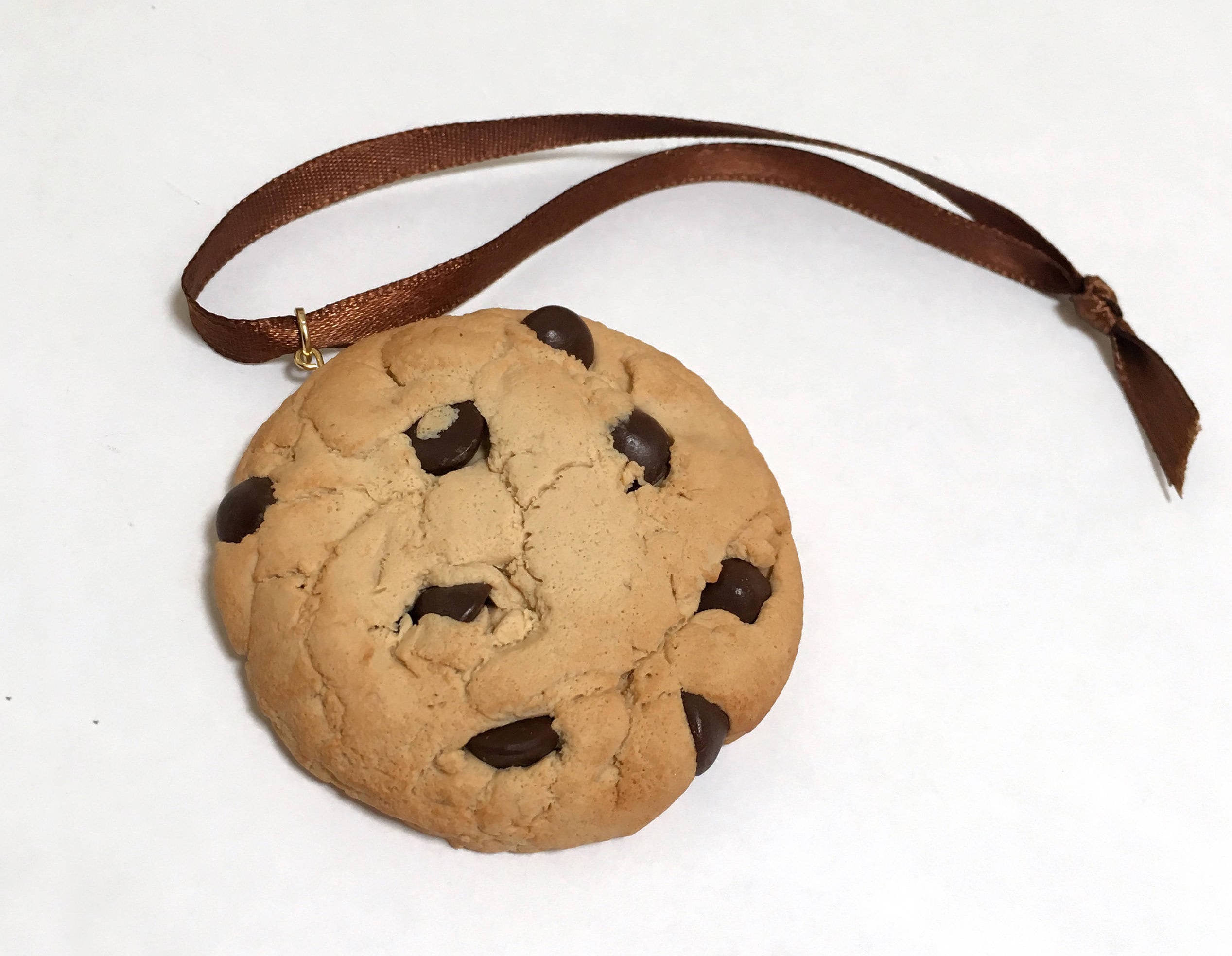The image depicts a hyper-realistic pendant designed to resemble a golden brown chocolate chip cookie, set against a stark white background. The cookie pendant features eight dark brown chocolate chips scattered across its surface, making it strikingly lifelike. A brown ribbon, which has a subtle shine, threads through a clasp at the top of the cookie and is tied in a knot, with two loose ends peeking out. The shadow cast by both the ribbon and the pendant adds depth to the image, accentuating the details of this delightful accessory.